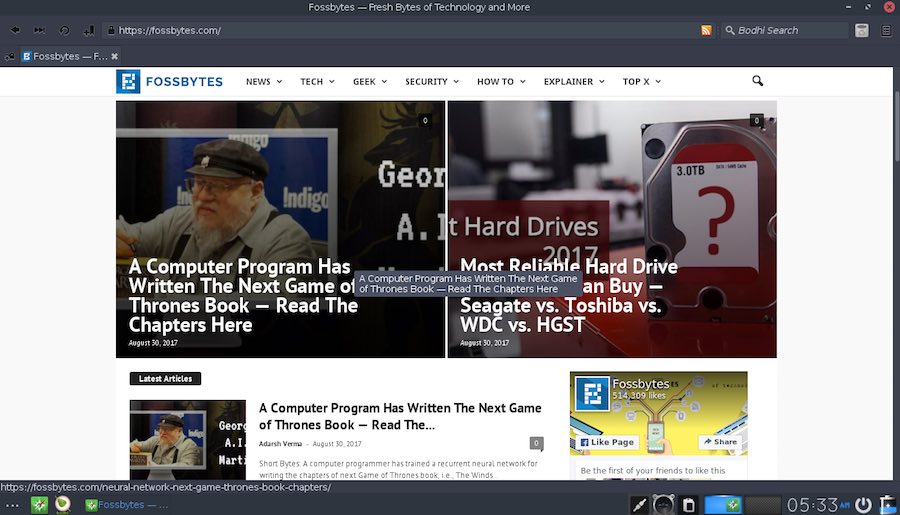**Detailed Caption:**

This is a screenshot of the Fossbytes homepage as viewed on a desktop. At the top left of the page, the Fossbytes logo is prominently displayed. Spanning the rest of the top area, there's a horizontal navigation menu featuring categories such as News, Tech, Geek, Security, How-To, Explainer, and Top X. Directly below this menu, two large square thumbnails are centered. 

The left thumbnail showcases an image of George R.R. Martin, the author of the Game of Thrones books, accompanied by text that reads, "A computer program has written the next Game of Thrones book, read the chapters here." The right thumbnail features an image of various hard drives with a text overlay stating, "Most reliable hard drives you can buy: Seagate vs Toshiba vs WDC vs HGST."

Additionally, there is a blue bar pop-up that spans over the center of both photographs, reiterating the message from the left thumbnail, "A computer program has written the next Game of Thrones book, read the chapters here." This bar partially obscures the images underneath it, drawing attention to the highlighted feature on the homepage.